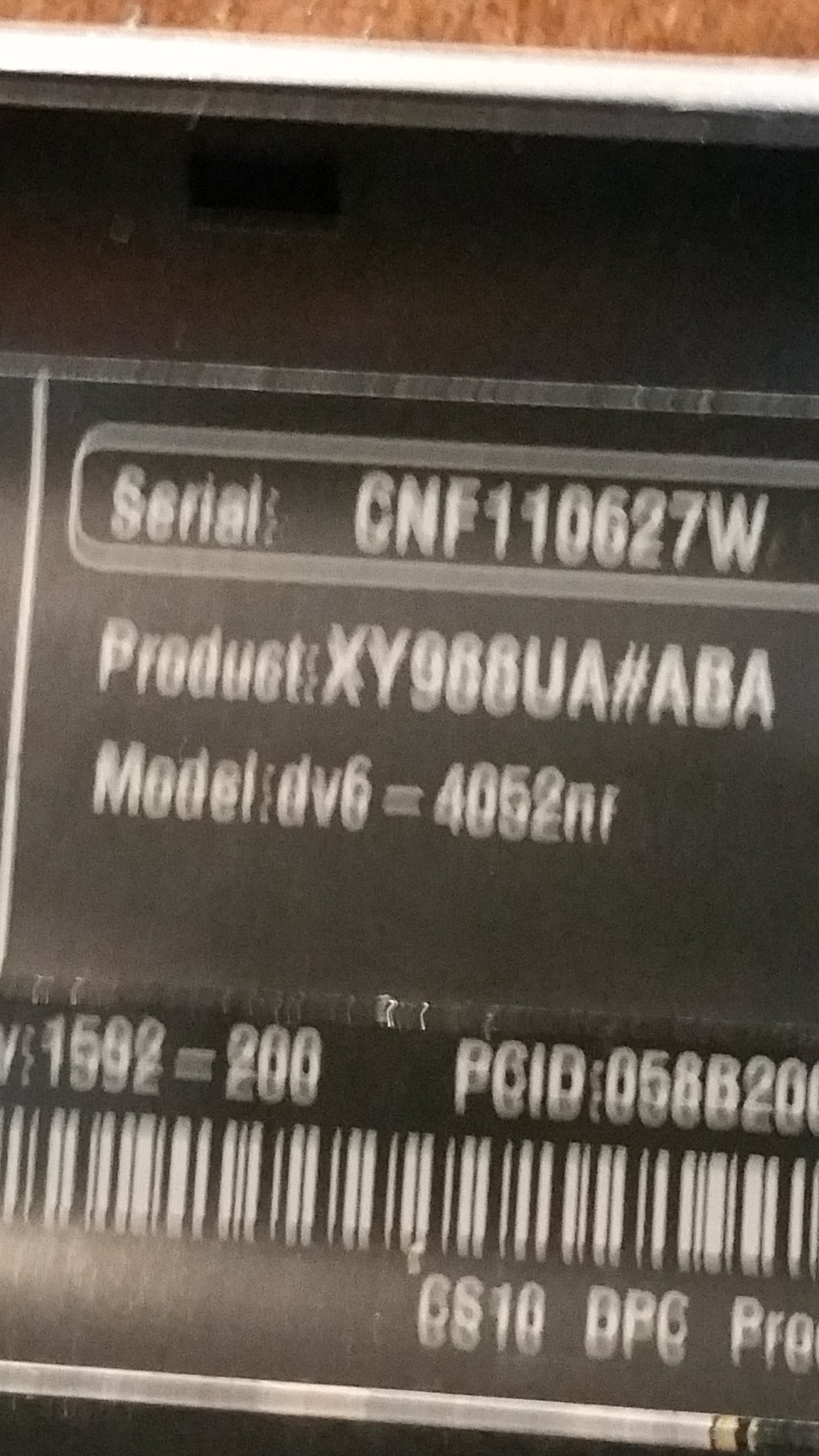The image captures the detail of a black label affixed to a rectangular black object. The label, featuring white text, is prominently displayed within the frame. A strip of brown wood and a strip of white, likely parts of a desk or similar surface, intersect the top edge of the photo. Another object, possibly a laptop or charger, is partially visible in the upper portion of the image.

The label itself is detailed with various pieces of information. At the top, a rectangular box with rounded corners contains the serial number "CNF110627W." Directly beneath this, the product code "XY988, UA#ABA" is displayed. Following that is the model number "dv6-4052nr," written in lowercase letters.

Further down, there's a traditional black-and-white barcode, and to the left of it, the number "1592-200" is printed. Above the barcode, the PCID number "058820" is partially visible but extends out of the frame.

In the bottom right corner of the label, the text "CS10 DPC PRO" is displayed, providing additional identification details. The meticulous arrangement of numbers and codes suggests this label belongs to a piece of electronic equipment, likely for inventory or identification purposes.